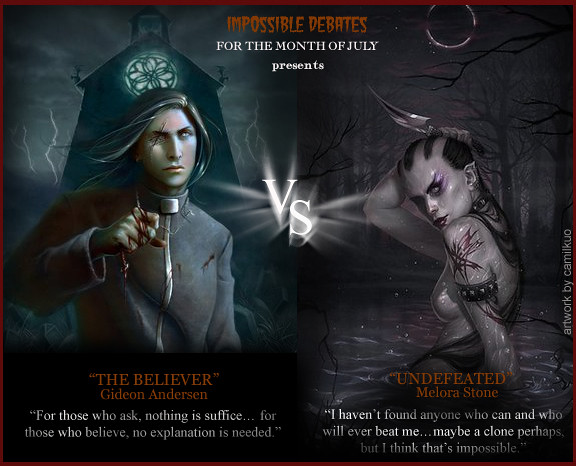This image appears to be a dark, atmospheric poster for a fantasy game or series, titled "Impossible Debates for the Month of July." The scene is set at night, with a leafless forest in the background. On the left side, a gothic church towers ominously. In front of the church stands a man with long hair, a futuristic Nehru jacket, and a pronounced scar traversing his right eye. His hand is bloody, or perhaps he is holding something bloody. This character is labeled as "DeBeliever, Gideon Anderson." On the right side, emerging from a dark, swampy lake beneath an eclipse, is a female figure with tattoos, long hair, and a dagger in hand. This character is referred to as "Undefeated, Meloria Stone." Both figures are digitally rendered, suggesting a high fantasy or gaming context. Text at the top announces the event, while additional white text provides further information about the characters. The artwork is credited to Camille Cool.